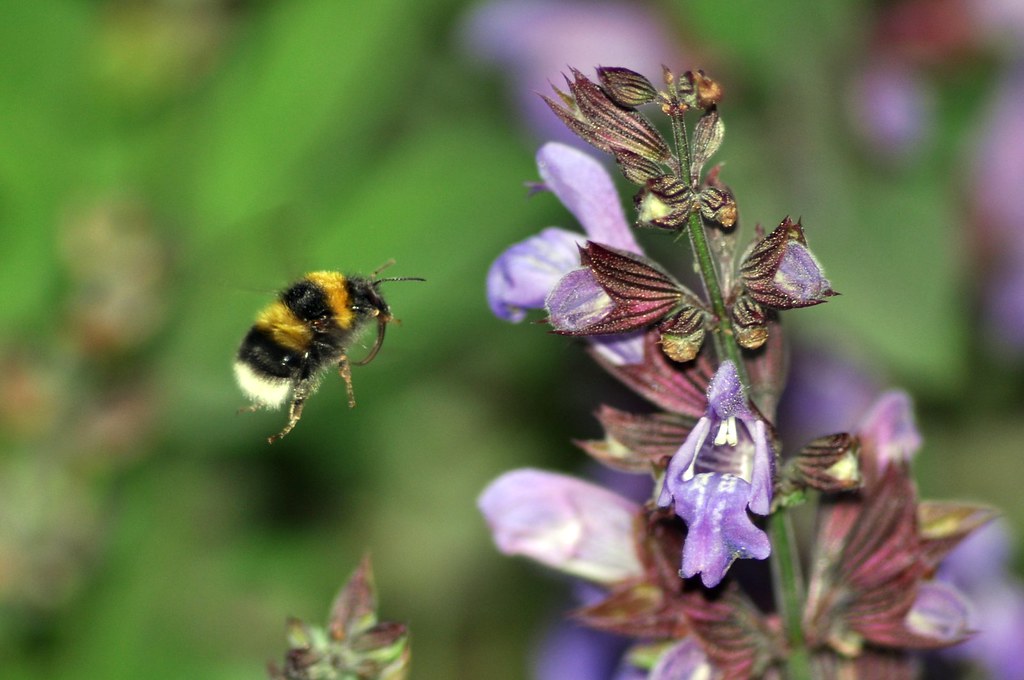In this vibrant photograph, we observe a bumblebee in mid-flight approaching a cluster of purple flowers. The bee, captured hovering in the middle-left portion of the image, displays distinctive black and yellow stripes, with a notable white stripe at the tail end. Its body appears pleasantly round and furry, dusted with grains of pollen on its legs and back, underscoring its active role in pollination.

To the right of the bee, a verdant green stem extends diagonally from the bottom right corner, adorned with multiple conical purple flowers, one of which is notably open and roughly the size of the bee itself. This open flower seems to be the bee's target, with its vibrant colors drawing the insect in. The background is intentionally blurred, creating a strong depth of field effect that ensures the viewer's focus remains on the dynamic interaction between the bee and the flowers. The overall setting is a picturesque scene of nature, emphasizing the crucial act of pollination.